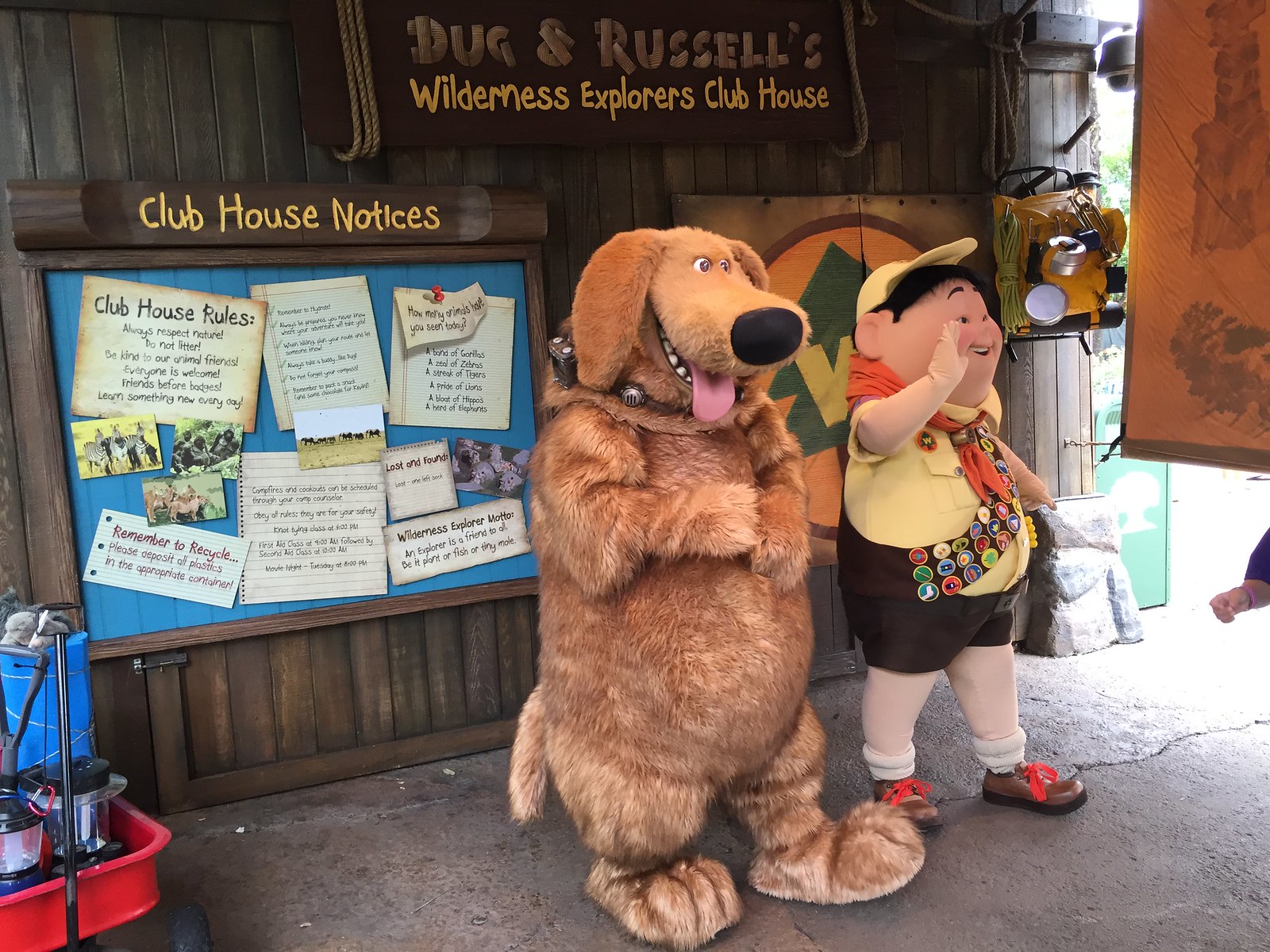In the photograph, two life-sized characters, both costumed, pose in front of a rustic, wooden wall. On the left stands a person in a large, brown dog costume with a playful expression, complete with a tongue sticking out. Next to the dog, on the right, is another character dressed as a young scout, adorned with a yellow shirt, black shorts, brown shoes, and a matching yellow cap. A sash filled with badges drapes across the scout's chest, signifying their many achievements. The background wall, made of dark brown wood, features two prominent signs. At the top, a sign reads "Doug and Russell's Wilderness Explorers Clubhouse" in bright yellow font, held up by a long piece of wood accented with ropes. Below, another section is labeled "Clubhouse Notes," showcasing a bulletin board cluttered with various paper notes like "Clubhouse Rules" and reminders to recycle, indicating a well-used and cherished space. This whimsical setup suggests they are likely at an amusement park, bringing a magical, make-believe world to life.